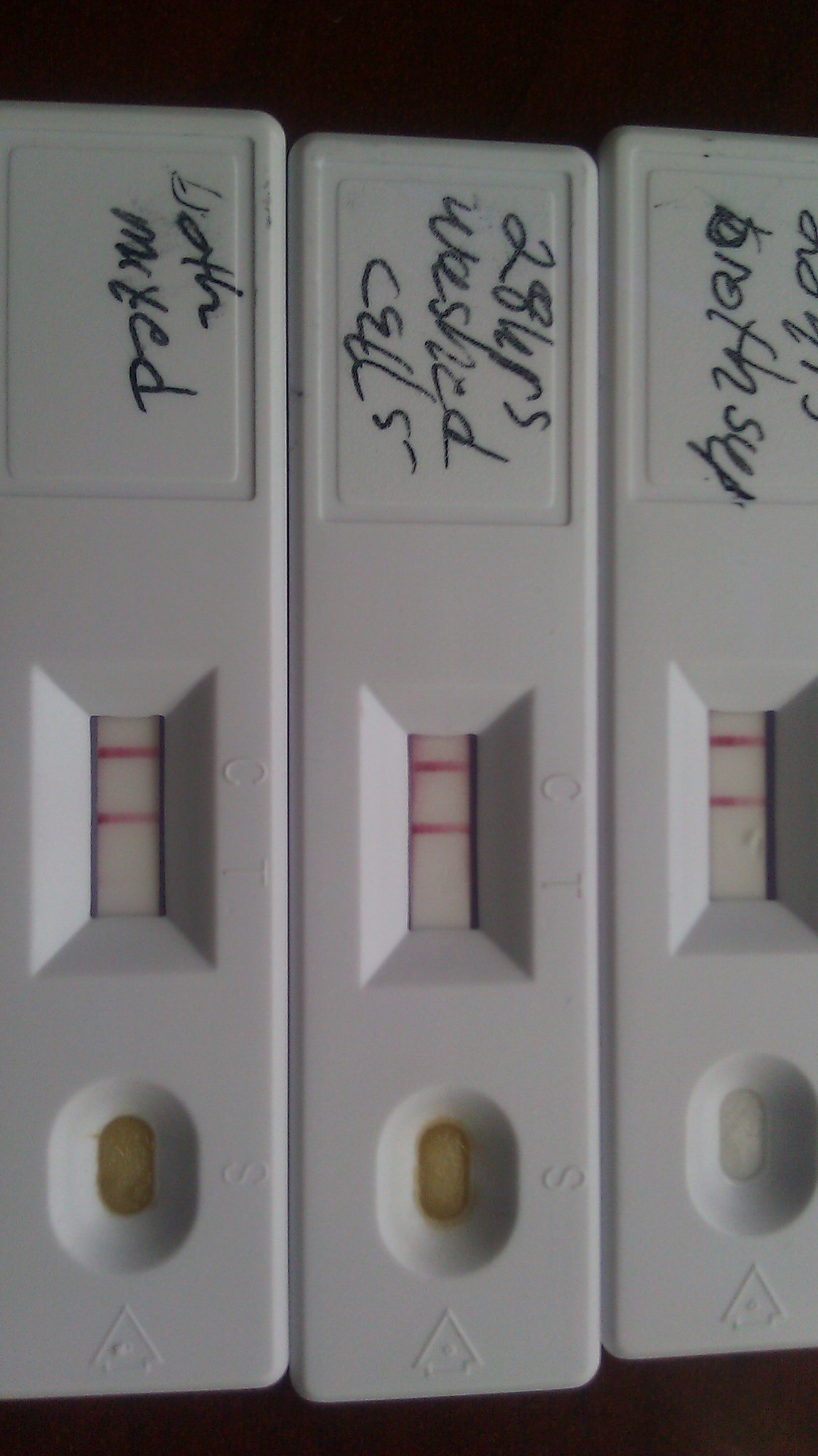The image captures three positive pregnancy tests, each intricately detailed with handwritten notes on their white plastic casing. The tests, featuring the standard design, exhibit an arrow directing where the sample should be applied, followed by two distinct windows for the control and test lines. Set against a stark black background, the pregnancy tests display the telltale pink lines indicating positive results, with a yellow tint where the sample is placed. Despite bearing a resemblance to COVID-19 tests, these pregnancy tests are distinguishable by their specific markings and structure.